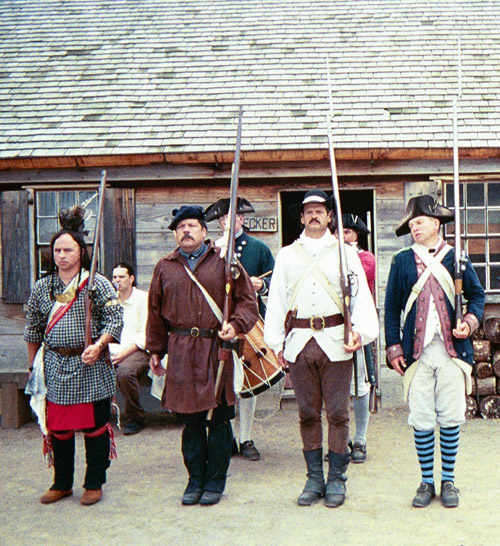In front of an old-fashioned house with wooden boards and grayish roof tiles, seven men are positioned in two rows, participating in what appears to be a historical reenactment of an American colonial period, featuring Native Americans, pioneers, and soldiers. The man on the far left is dressed in Native American attire, with his hair up in braids, adorned with a feather headdress, red ribbons tied around his knees, a black and white checkered shirt, and black pants. Next to him, a man wears a light brown trench coat and a beret, paired with black pants, and has a mustache. The third man dons a white coat over a white undershirt, brown pants, and a brown belt with a gold buckle. The fourth man, possibly dressed to resemble a Revolutionary or Civil War soldier, is in a blue shirt and white pants with knee-high white socks and is carrying a musket. 

Behind these men, another row features figures dressed in historical European military garb. One man in a green overcoat with brass buttons, a white collar, white stockings, and a three-point hat holds a drum. Nearby, another in brown pants, black boots, and a white overcoat with a brass-buckled belt also carries a musket. Toward the right, a man in a three-point hat and red coat with a white collar, wearing white pants and light blue stockings, stands with a musket. The far-right figure sports a blue overcoat with red trim, white pants, striped socks, and brown shoes. The house in the background features a partly visible sign with the letters "E-C-K-E-R," adding to the atmosphere of the historical setting. The scene is filled with shades of black, white, gray, blue, red, yellow, and tan, capturing the essence of the reenactment.